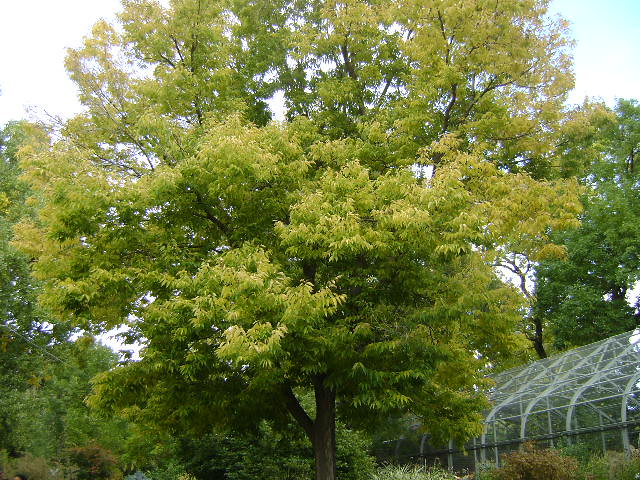The color photograph captures an outdoor scene centered around a tall, deciduous tree with a brown trunk and lush, rounded foliage composed of mostly green leaves with some yellow. The tree stands prominently in the middle of the image, surrounded by an assortment of trees and shrubs, both green and brown. In the lower right-hand corner of the image, there is a clear glass greenhouse framed in light silver metal. The greenhouse appears domed and arched, with no reflection of the sun visible on its surface. The background reveals a blue sky with scattered wispy white clouds, contributing to the bright and fairly clear day. The scene is set in a natural wooded environment, with ornamental grasses and shrubs contributing to the layered, textured landscape.